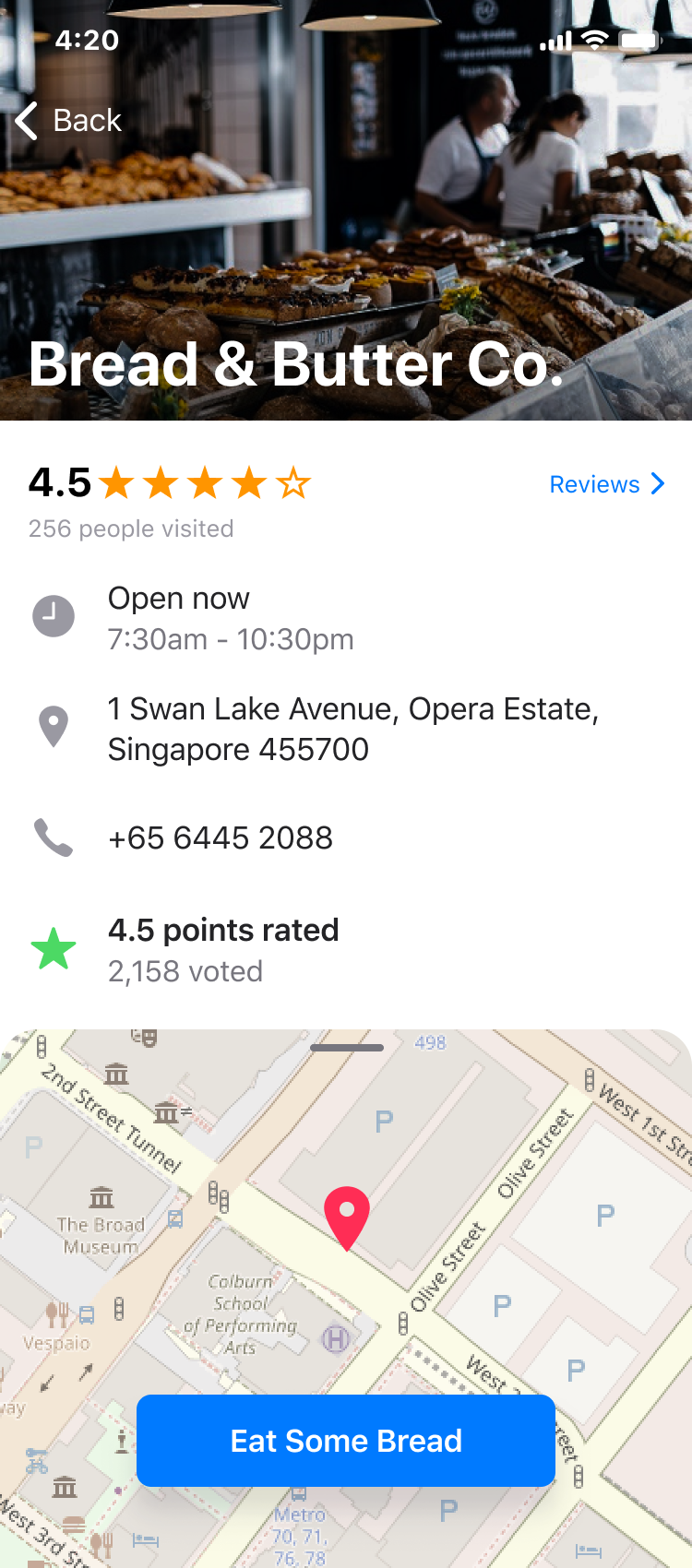This colorist screenshot from a website showcases a detailed overview of a mobile phone interface. At the very top, the time is displayed in white as "4:20." To the left, various mobile icons are visible, while the right-hand corner shows WiFi and signal strength indicators.

On the left side of the screen, there is a back arrow with the word "Back" written underneath. The main image captures a quaint bakery setting, labeled "Bread and Butter Co." in white text at the bottom. Two individuals, likely bakers, are seen working in front of a large window, with numerous shelves of freshly baked goods behind them. The bakery is illuminated by two overhead lights and features a right-side window view.

Below the image, a white background with black text provides detailed information about the bakery. It boasts a rating of 4.5 stars and indicates "Reviews" in blue, noting that 256 people have visited. The bakery is "Open now," with operating hours from 7:30 AM to 10:30 PM. The location is specified as Gwan Swan Lake Avenue, Opera State, Singapore, 455700, with the contact number 6564452088. A second rating section highlights that 2168 users have voted, represented by green stars, contrasting with the orange stars above.

At the bottom, a map pinpoints the bakery's location, showing nearby diamond-shaped roads and building blocks. The center of the map features a blue label with white text that reads, "Eat Some Bread."